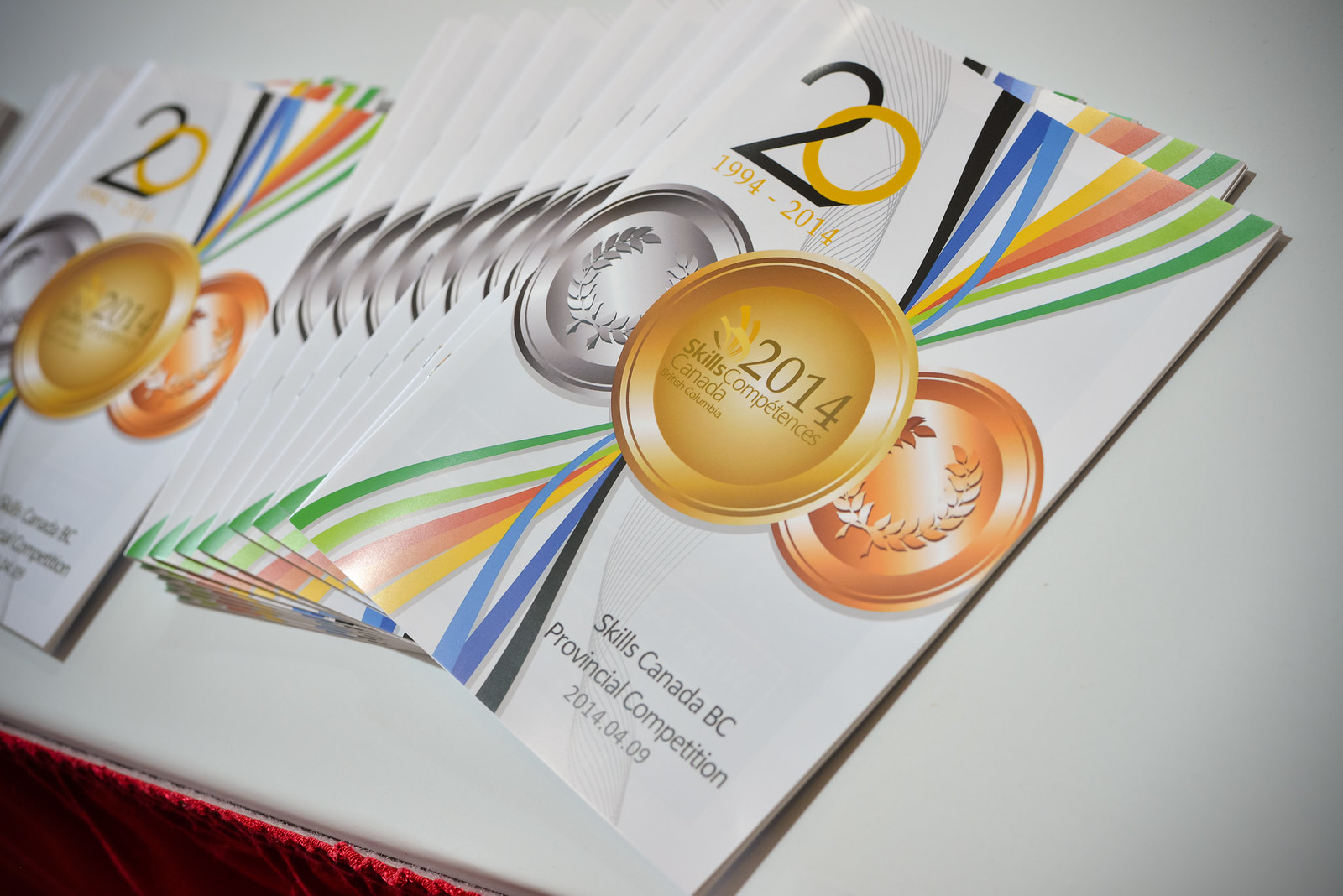The image features an indoor setting with a table adorned with a tablecloth and table skirt, prominently showcasing neatly fanned out stacks of identical brochures placed centrally. These brochures are for the 2014 Skills Canada BC Provincial Competition, featuring a dynamic and vibrant cover design. At the top left corner of the brochure, the number "20" is displayed with the "2" in black and the "0" in orangey-yellow, followed by the years "1994 to 2014" in yellow lettering. The centerpiece of the brochure highlights gold, silver, and bronze medals, with the gold medal prominently displaying the text "2014 Skills Competences Canada, British Columbia." Below the medals, various colorful ribbons—black, blue, yellow, pink, white, and shades of green—cascade from the top to the bottom of the page. Additional text at the bottom right corner reads "Skills Canada BC Provincial Competition 2014-04-09." The brochures, predominantly white with multicolored accents, are arranged in multiple layers, suggesting a quantity of 20 to 30.